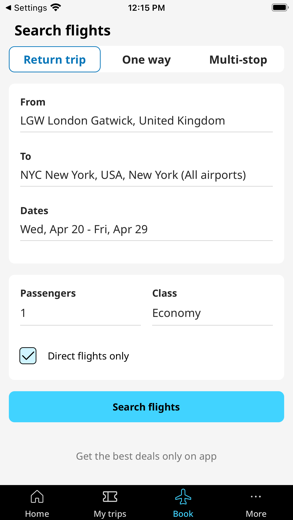This image is a detailed screenshot of a cell phone displaying a flight search interface. In the upper left corner, the status icons show the settings, Wi-Fi connectivity, the current time of 12:15 p.m., and a full battery indication. Below, in bold black text, it reads "Search flights."

Directly underneath, there are three buttons arranged side by side: "Return trip" highlighted in blue text, "One-way" in black text, and "Multi-stop" also in black text. The flight itinerary is specified in a white box below these buttons, showing the departure airport as "LGW London Gatwick, United Kingdom" and the destination as "NYC, New York, USA (all airports)."

The travel dates are listed as "Wednesday, April 20th" to "Friday, April 29th." Below this, details about the passengers and travel class are provided: "1 passenger, Economy class." There is also an option checked off in a light blue box for "Direct flights only."

At the bottom of the screen is a prominent blue action button with the label "Search flights" in black text.